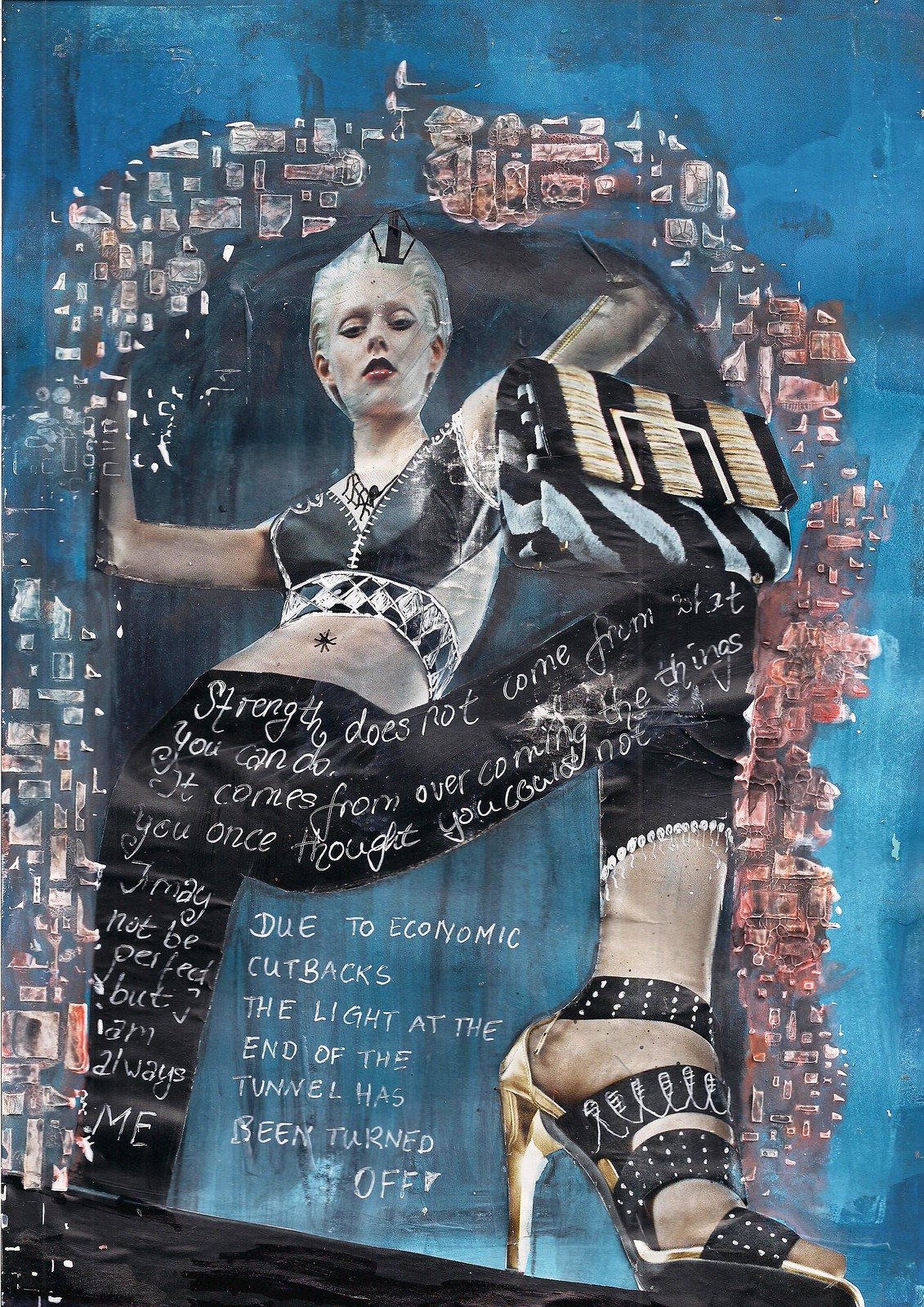The image depicts a hand-painted artwork set against a deep blue background, featuring a young woman with short blonde hair and red lipstick. She is dressed in a black and white halter top exposing her midriff, and tight black pants bearing a motivational text that reads, "Strength does not come from what you can do, it comes from overcoming the things you once thought you could not." In addition, her posture is striking, with her left leg elevated onto a ledge, showcasing her high-heeled black shoes with gold heels. Below her leg, an additional piece of text solemnly states, "Due to economic cutbacks the light at the end of the tunnel has been turned off." The woman appears to be emerging from a hole in the wall, drawing the viewer’s focus with her bold and confident stance at the center of the image. The use of vibrant colors like black, white, tan, gray, gold, brown, pink, red, yellow, and purple adds dynamism and depth, reinforcing the powerful message conveyed through the artwork.